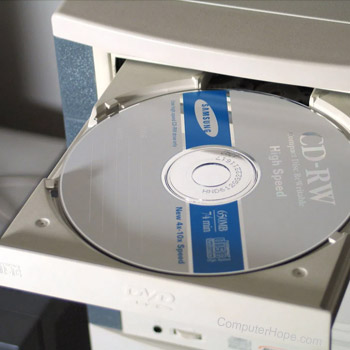The image depicts a CD/DVD drive tray extended from a tower computer. The drive, which is embedded in a beige tower with a gray strip down the left side, has the word "DVD" in raised lettering on the front near the bottom. The drawer, appearing white with gray elements, is fully open, revealing a CD-RW disk branded by Samsung. The disk is primarily silver with a dark blue stripe across the middle and the text "CD-RW" in silver on the top, facing the right side. The area around the center of the disk is transparent. The photograph, taken from an overhead angle, presents a clear, detailed view of both the tray and the disk, emphasizing the color contrasts and the realistic textures of the materials.